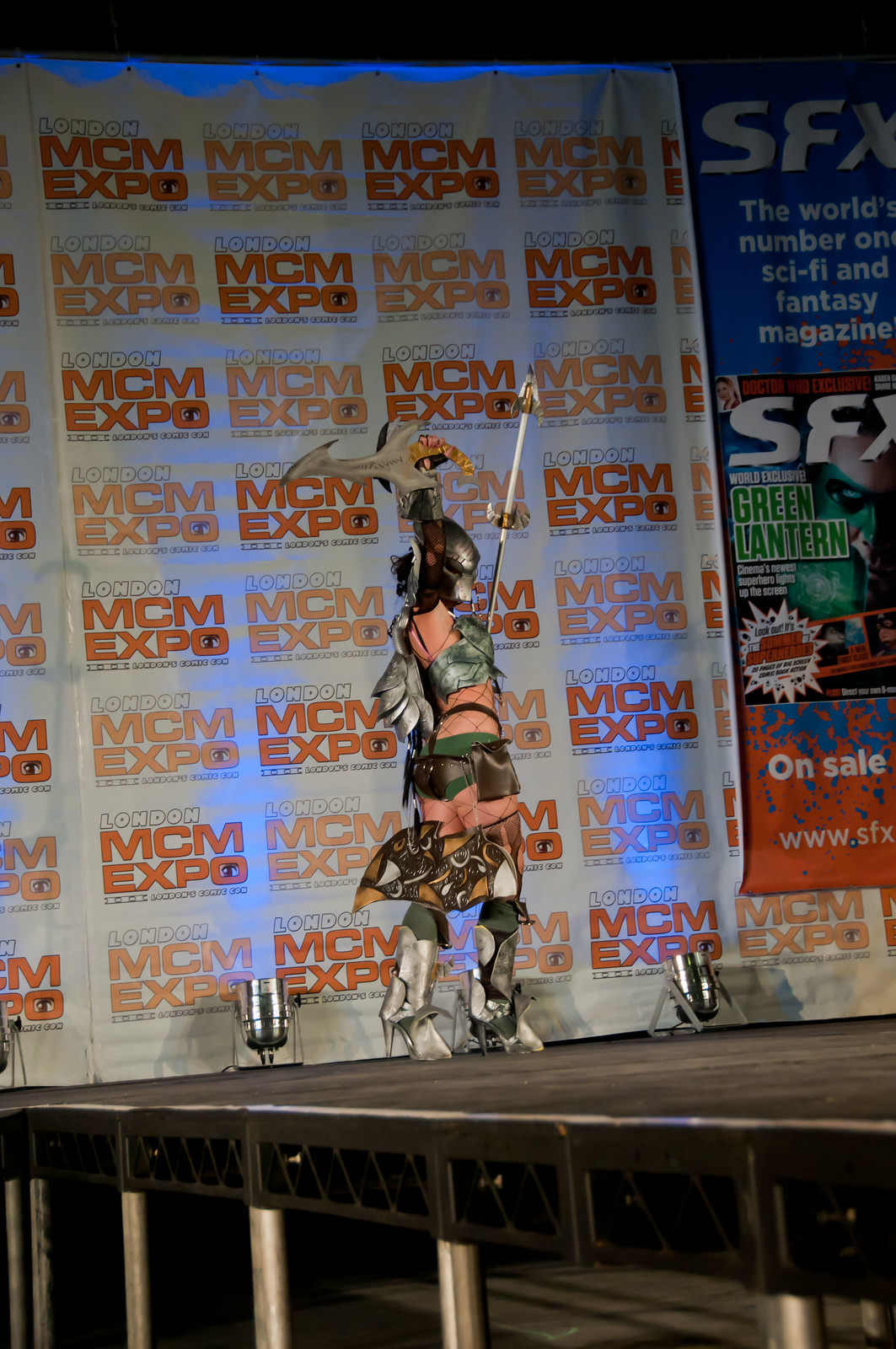This is a detailed color photograph taken at the London MCM Expo 2002, capturing a female cosplayer standing on a stage adorned with banners repeatedly showcasing the event's logo. The stage is slightly elevated, allowing a view of its metal supports and the performer at foot level. The woman is fully immersed in her character, donning an intricately designed metallic helmet and visor that covers her entire head and face, evoking the iconic look of the Predator. She wears a dark green bikini top and matching bottoms, accompanied by a belt around her waist. Her outfit is complemented by knee-high green socks and striking silver high-heeled boots. Noteworthy are the razor-sharp wing-like attachments projecting from her thighs and the wing-like apparatus on her back. Completing her ensemble is a messenger pouch around her hip and a long spear-like scepter in her hand. She stands confidently between two bright spotlights on the stage, her pose emphasizing the elaborate homemade weaponry and armor that include a chest plate with no underlying shirt. The right side of the background prominently displays an ad for "SFX, the world's number one sci-fi and fantasy magazine," amidst various other sci-fi themed advertisements.